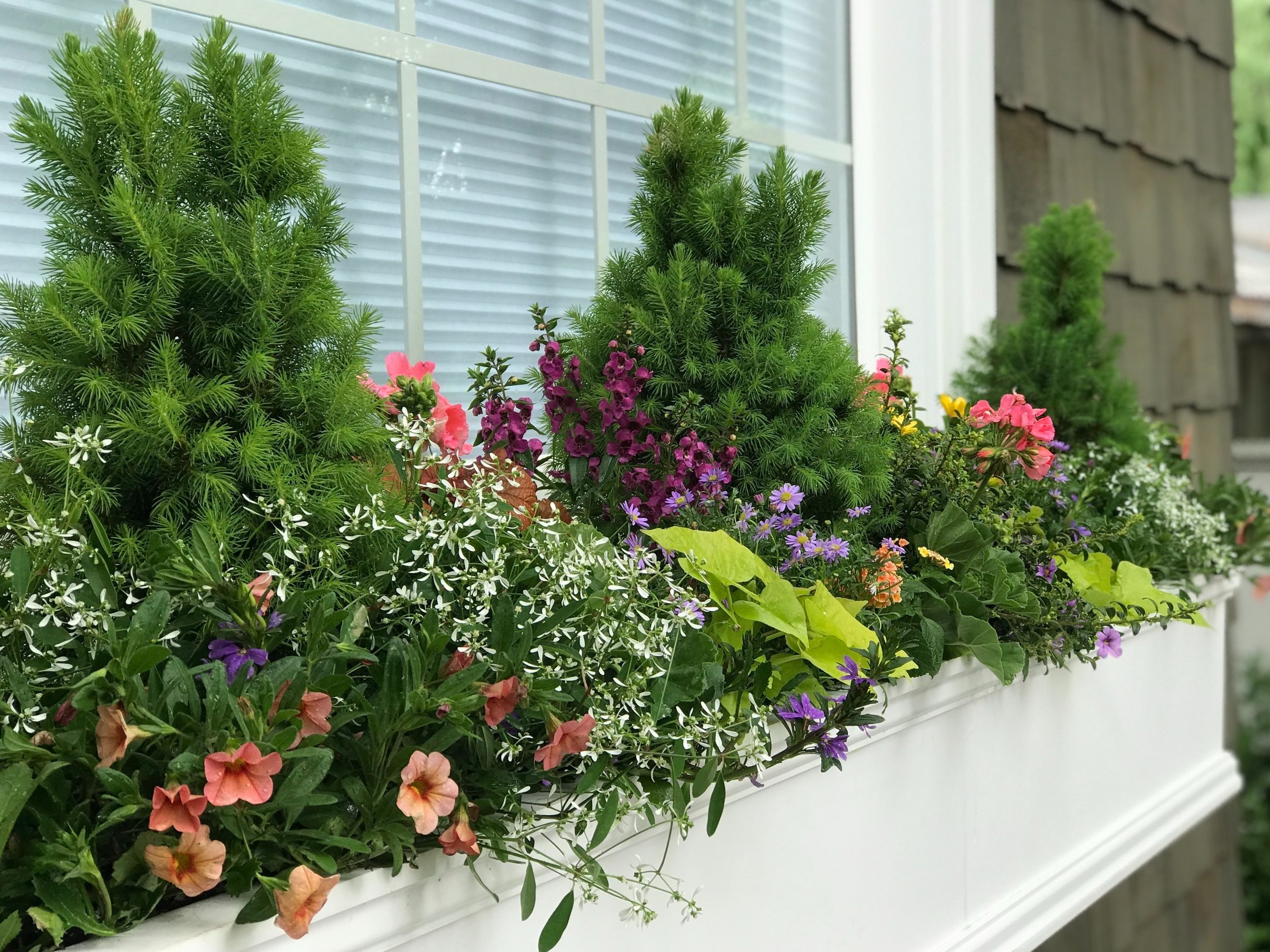This photograph captures a charming windowsill garden located on the exterior of a house. The green wall of the house provides a lush backdrop for the meticulously arranged rectangular white planter boxes, which feature ornate trim along their edges. The windows behind the planters, adorned with closed blinds and cheap shutters, frame the composition nicely.

Each planter box brims with a diverse assortment of flora. Standing tall are small pine shrubs, lending a touch of evergreen to the scene. These are complemented by a colorful mix of flowers, including pink tulips, purple lavenders, and small white flowers. Additionally, there are vibrant orange and yellow blossoms, all creating a vibrant, harmonious palette.

The planter boxes are positioned on a white windowsill, which, despite appearing spacious, is filled to the brim with this verdant display. On the upper right quadrant of the image, the wall transitions to a brownish stucco texture. The lighting in the photograph is excellent, emphasizing the vivid colors of the plants and the details of the ornate planters, though it is unclear if the scene is under direct sunlight or an overcast sky.